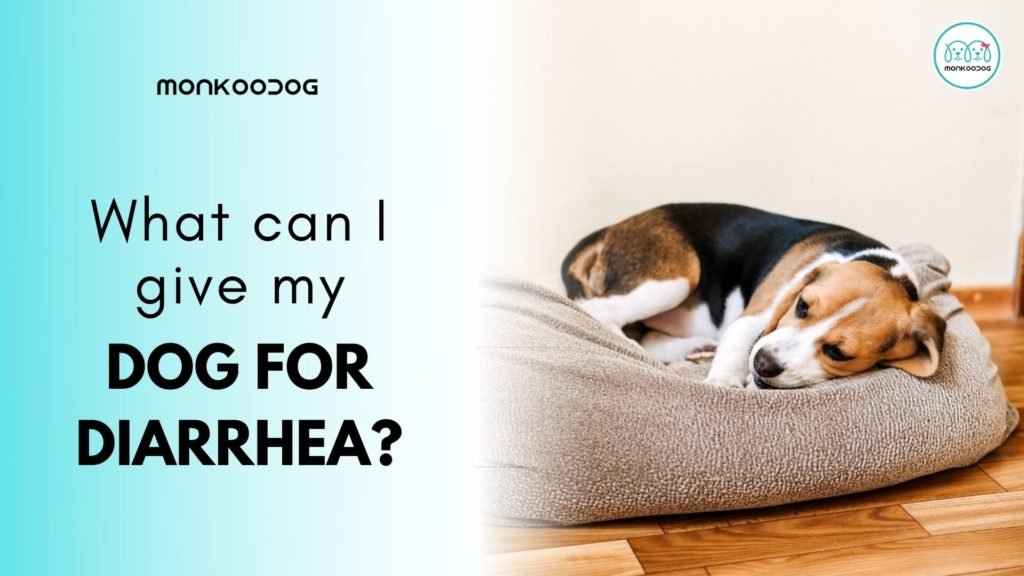In this image, a beagle puppy, featuring a brown nose, white facial markings, brown hair on its head, and a coat that is a mix of black and brown, is curled up in a gray dog bed. The bed is situated on brown hardwood flooring. The pup seems to be resting or perhaps a bit downcast. On the left side of the image, against a backdrop that transitions from mint green to turquoise, there's prominent text in black which reads, "What can I give my dog for diarrhea?" with "Dog for Diarrhea" in bold, uppercase font. Above this text, there's a logo reading "Monkoodog" in black, accompanied by an image of two dogs, one adorned with a pink ribbon. The same Monkoodog logo, featuring the word and the two dogs, also appears in the upper left and upper right corners of the image.